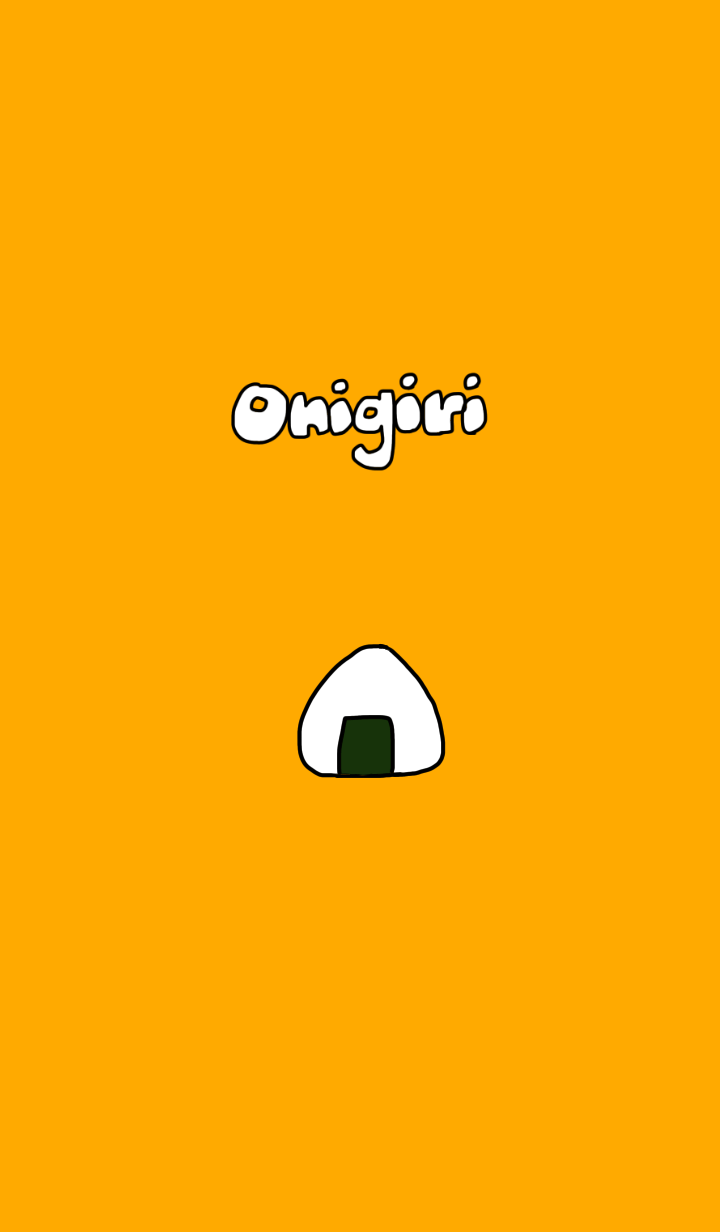The image features a muted tangerine-orange rectangular poster with a cartoony design. Dominating the upper middle section of this long rectangle is the word “Onigiri” written in a bubbly, modern font. The letters are white and outlined in black, making them appear hand-drawn and somewhat smooshed together. Below this text is a simple, cartoony depiction of an Onigiri: a white, rounded triangle representing rice, with a small, black rectangle at its base symbolizing a piece of seaweed. The Onigiri image is outlined in black, and together with the text, it forms a minimalist and playful composition against the muted orange background.